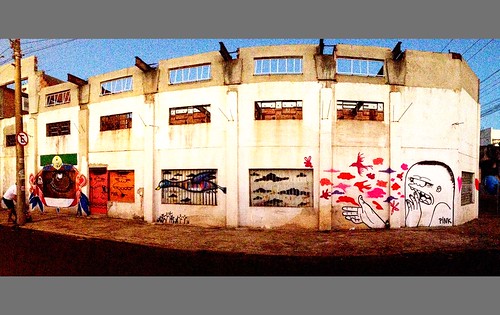The image captures a wide-angle view of an old, abandoned factory situated on a street corner, prominently featuring a vivid blue sky above. Dominating the scene is a three-story, roofless, concrete building with its white facade extending three-quarters of the way up before turning brown at the top quarter, punctuated by square holes with bars descending from them. Numerous windows, some of which are boarded up, are visible, each adorned with distinct pieces of graffiti art, transforming the dilapidated structure into a canvas of color and creativity.

To the left side of the building, a man in a white shirt and blue jeans stands next to a telephone pole bearing a sign, seemingly engaged in the act of creating graffiti. The art under the first window features a whimsical figure with blue hair and a prominent facial feature that could be interpreted as either a large nose or a broad smile. The second window displays an orange background with two faces, one on a door and the other on the window, characterized by exaggerated teeth. The third window showcases a green duck or goose with a red torso and background clouds, which extend into the fourth window as more black clouds. The final window features an imaginative scene of birds being blown across by a creature with an eraser-like head, further enhanced by red clouds and more red birds above.

This captivating scene blends the desolation of an abandoned structure with the vibrancy and creativity of graffiti, challenging the conventional notions of urban art as mere graffiti by presenting it as a cohesive and intricate mural that breathes new life into the decaying factory.